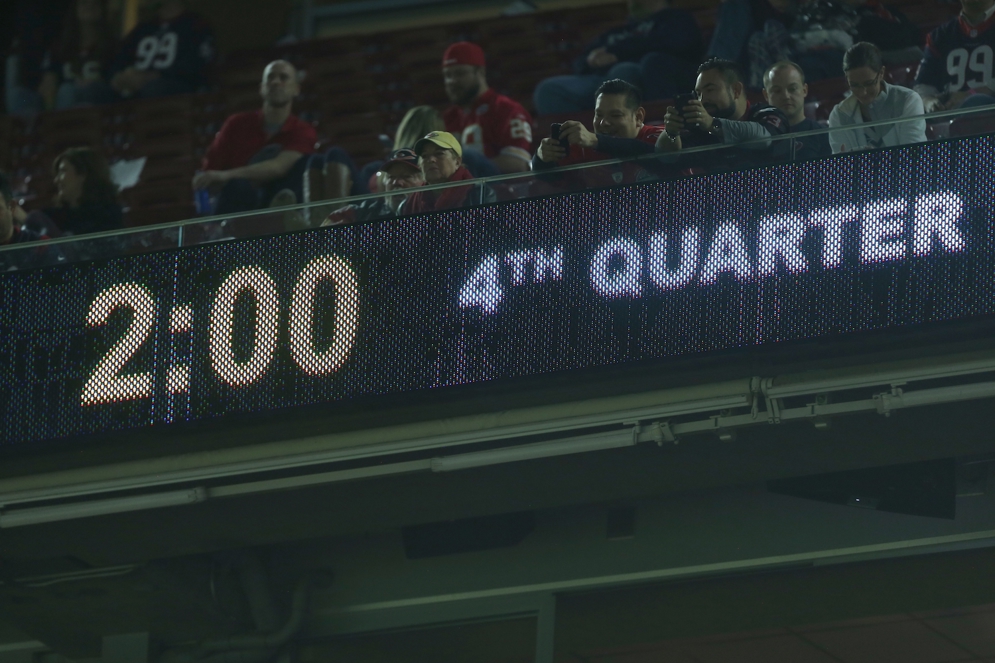The image captures a moment at a football game, focusing on a digital sign indicating "2:00" in yellowish letters and "Fourth Quarter" in white letters. The sign is situated among the upper deck seating, where you can see a small section of fans dressed in football jerseys. Although it is not well lit, the image is clear, emphasizing the excitement of the last two minutes of the fourth quarter. Some seats in this section are empty, accentuating the intensity among the scattered fans who are intently watching the game. The overall color photograph zooms in on the sign and surrounding fans, omitting the field and players, giving a tight, detailed glimpse into this critical moment of the game.